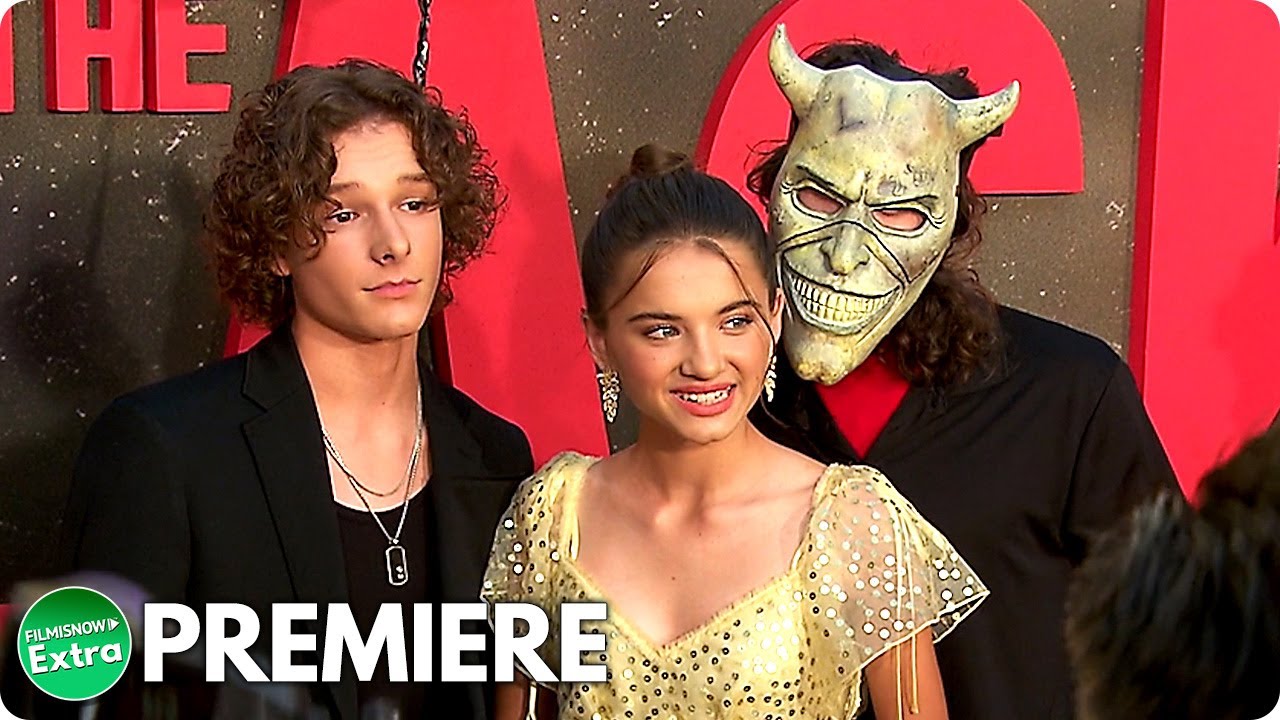This YouTube thumbnail appears to be from a channel called FilmSnowExtra, as indicated by the green logo and the word "Premiere" in white text positioned in the lower left corner. The image is a close-up, outdoor photograph captured at a movie premiere, featuring three individuals prominently in the center frame. 

On the left is a young man with brown, curly hair, dressed in a black jacket and wearing a dog tag around his neck. In the center stands a young girl, possibly around 15 or 16 years old, wearing a yellow polka-dotted dress with her hair pulled back in a bun, also adorned with earrings. She is smiling and looking off to the left. Behind her to the right is another young man, dressed in a red t-shirt and a red tuxedo. He is wearing a distinctive uncolored or brownish devil mask with horns and a grinning expression. The trio stands in front of a nondescript billboard featuring some indecipherable red lettering.

Combining elements from all descriptions, this detailed caption captures the essence and specifics provided by all contributors.